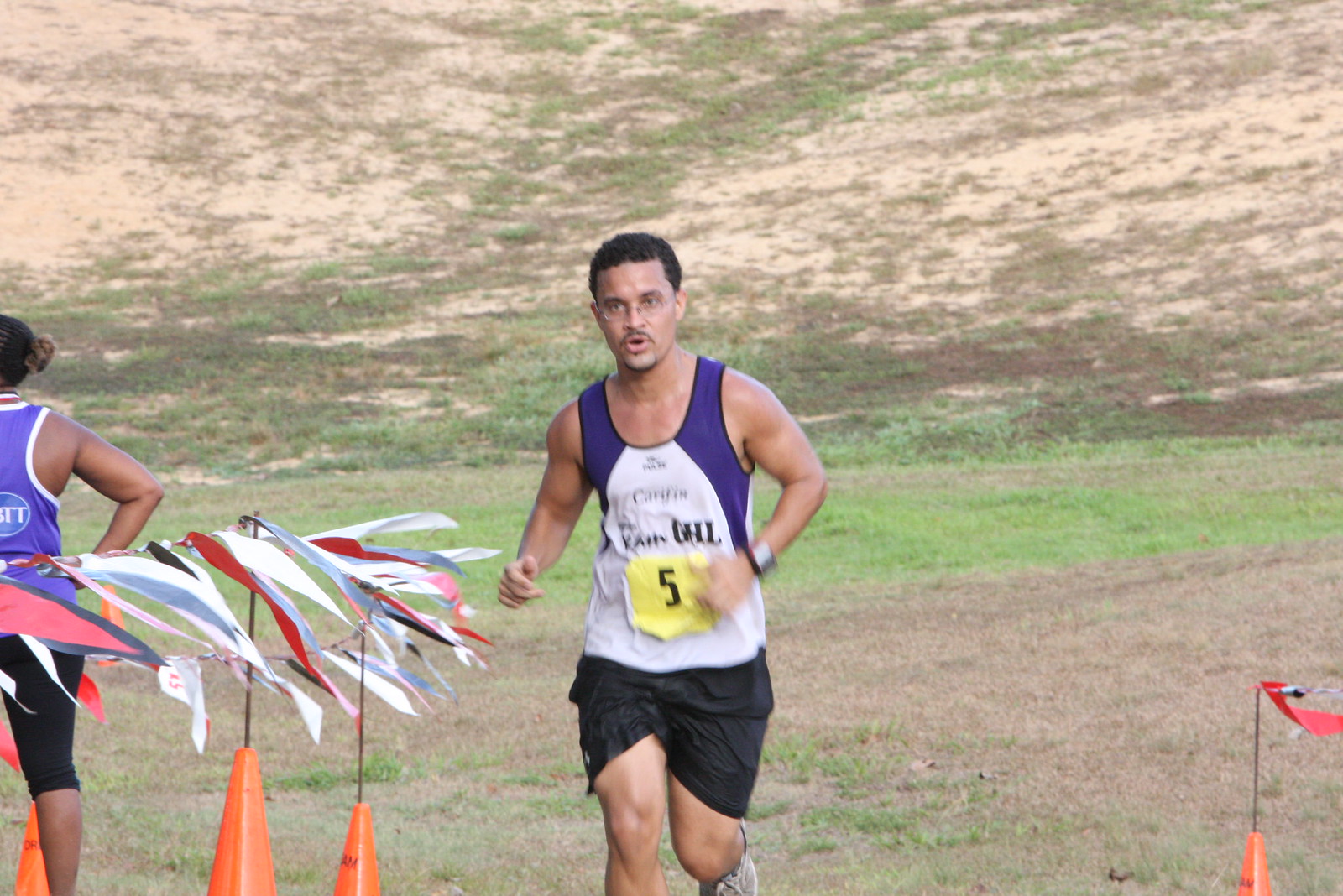This photo captures a high-energy moment during a marathon, featuring a central male runner with short, curly, dark hair, and a half-goatee beard. He is wearing wire-rimmed glasses, a purple and white athletic running vest, and black shorts. His race number, a prominent yellow "5," is pinned to his chest near his belly button. His heavily muscled legs are in full stride as he runs through a lineup of orange cones adorned with plastic pennants, suggesting he is close to the finish line. The ground is a sandy beige color with moderate tufts of grass. To the left and slightly behind him, a female runner is visible from the back. She is wearing a purple vest and long lycra-type cycling shorts. As a black woman, her right arm and leg are discernible, adding context and movement to the scene. The photo's vivid colors include orange, red, yellow, blue, black, green, and sandy beige, enriching the dynamic and competitive atmosphere of the marathon.